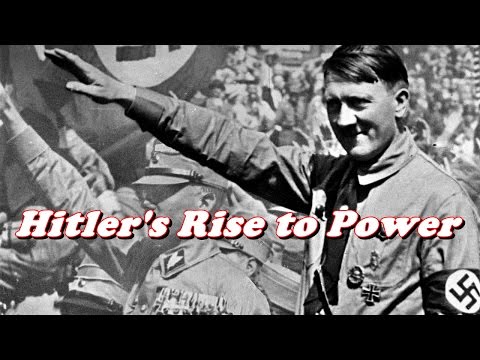This is a black and white poster or photograph of Adolf Hitler, prominently positioned in the front with an expression marked by an unsettling grin. He is seen squinting in bright sunlight with his right arm extended forward in the Nazi salute, while his left arm bears the distinct Nazi armband. Hitler is also adorned with three metal clips on his left side. Behind him, a row of Nazi officers stand in similar salutes, and a large crowd is visible further in the background. The image is slightly blurry, yet one can clearly see the white letters with red outlining across the center, stating "Hitler's Rise to Power." In the top left corner, a partially-visible Nazi flag displays a dark background with a white center and part of the Swastika emblem. The scene is set outdoors under a clear, sunny sky, casting a stark light that sharply defines the shadows.